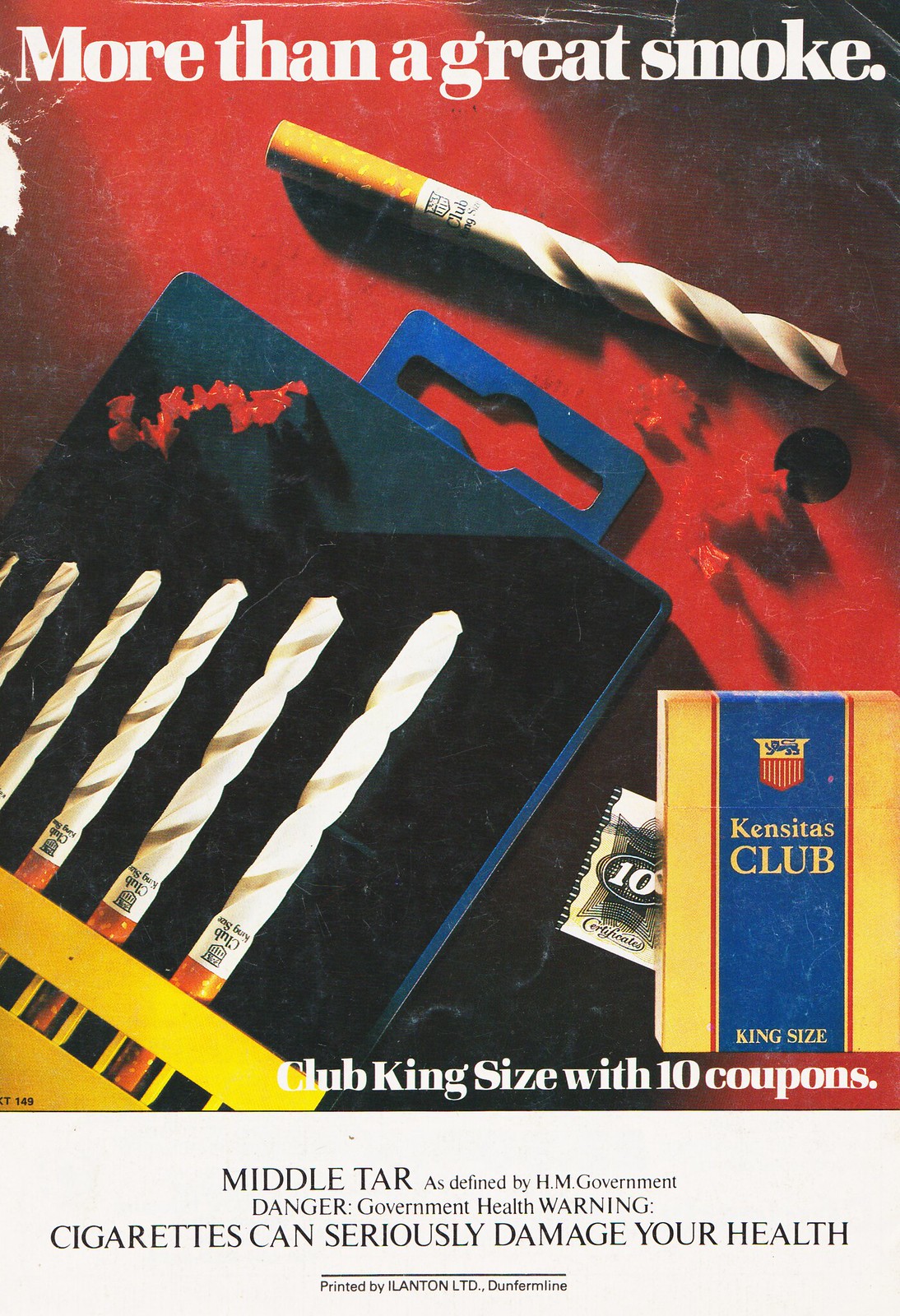This is a vintage advertisement for Concedus Club King Size cigarettes, printed by Layton Limited. The central image depicts a packet of cigarettes with one cigarette removed and laid out above the top of the container. The cigarette features a distinctive yellow filter and a crinkled, twisted white paper that makes it look like a drill bit. This drill-bit-like cigarette appears to have drilled a circular hole into the surface it rests on, resembling a drill bit holder.

In large white letters across the top of the advertisement, the slogan "More than a great smoke" is prominently displayed against a vibrant red and black background. Below this text, to the left, a black and blue label emerges, reinforcing the twisted appearance of the cigarettes. Positioned to the right, a gold and blue box is marked with "Concedus Club King Size" along with the offer "10 coupons."

At the bottom of the image, further descriptors read: "middle tar, as defined by Her Majesty's Government," and a health warning in white text against a white background cautions, "Cigarettes can seriously damage your health."